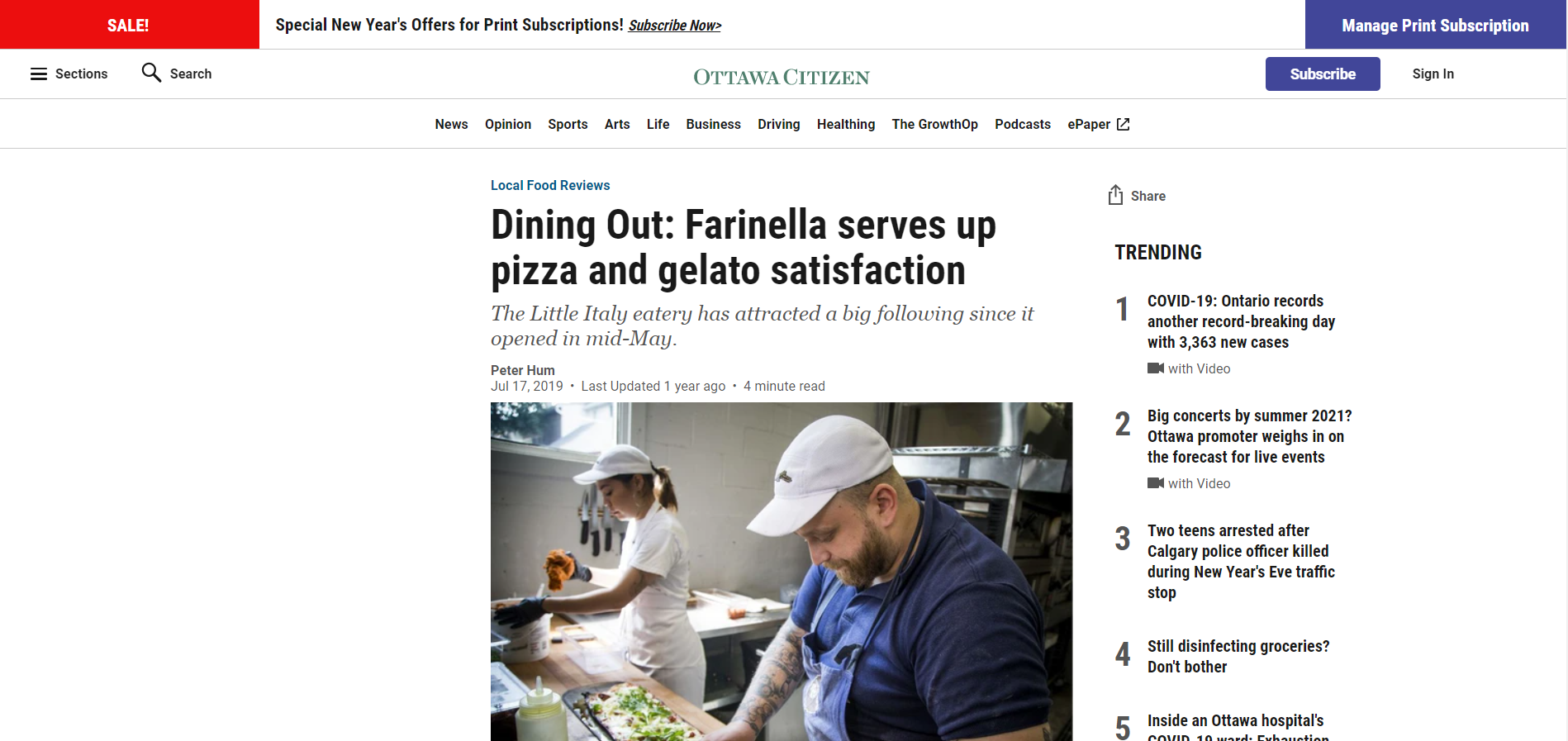### Detailed Caption for Newspaper Subscription Image:

The image captures a promotional ad from the Ottawa Citizen newspaper, prominently featuring a bold "Sale!" announcement at the very top, enclosed in a red box for emphasis, with an exclamation mark to convey excitement. The special New Year's offers for print subscriptions are detailed below, with an invitation to "Subscribe Now." The phrase "Subscribe Now" is underlined and appears as a clickable hyperlink. 

On the far right, there is a "Manage Print Subscription" button within a white context, outlined in a blue box. Below this, the "Ottawa Citizen" logo is displayed in green, capitalized letters. Adjacent to this logo, on the right side of the image, there is another blue "Subscribe" button and a black "Sign In" option.

Beneath the main header, a navigation menu spans the center of the image, listing categories such as News, Opinion, Sports, Arts, Life, Business, Driving, Healthy Living (though it appears as a single word "HealthyHealthy"), and additional categories like Podcasts and Paper.

A headline for a local food review titled "Dining Out" is featured prominently, highlighting an article that commends Parnelli's for its pizza and gelato offerings. Below this, the image highlights two individuals preparing food. One, an Asian woman with a ponytail wearing a hat, white apron, and white pants, is holding and seemingly smashing an ingredient with one hand. Beside her, a man donned in a white hat and blue apron is also engaged in cooking activities.

To the right, under a "Trending" section, multiple headlines catch the eye, including an article about "COVID-19 Records Another Record-Breaking Day," a feature on summer concerts for 2021, and three other trending articles.